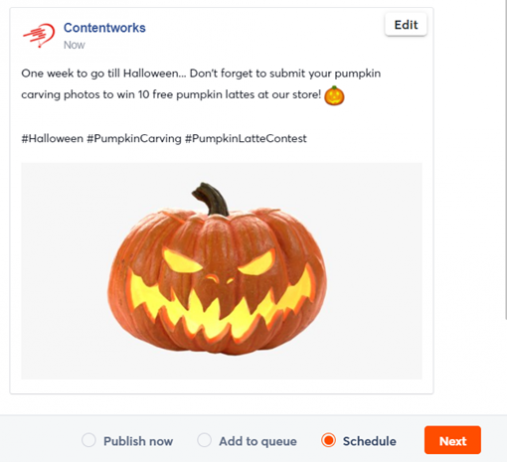In the image, we see the logo for "Content Works" prominently displayed in the upper left-hand corner in a unified blue font, with a capital "C" starting the word. Just to the left of the logo, there is a red symbol that resembles a harp, outlined in red with a clear middle. Diagonal lines extend towards the center of this harp-like symbol. On the upper right-hand side of the image is an "Edit" button.

Below the logo, a message reminds viewers: "One week to go till Halloween. Don't forget to submit your pumpkin carving photos to win 10 free pumpkin lattes at our store." This is followed by a pumpkin emoticon, two spaces, and a series of hashtags.

Finally, the lower part of the image features a picture of a carved pumpkin with an intimidating expression, showing sharp, mean-looking features with yellow eyes and a yellow glow emanating from its mouth.